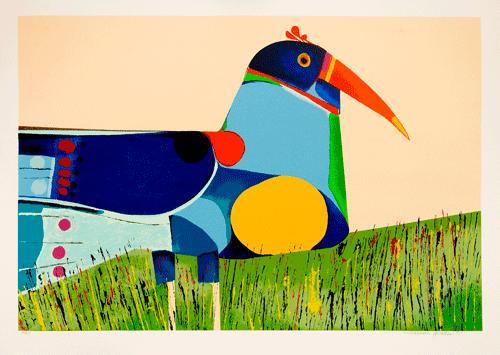This wide, rectangular painting, bordered by a thin, light beige frame, features an abstract or cubist representation of a colorful bird, reminiscent of a toucan. Positioned on the left side of the image, the bird faces right, set against a creamy vanilla or peach background that dominates the top half of the scene. The bird's head is dark blue with a prominent orange beak accented by yellow stripes and ends in a yellow tip. A crown of three red feathers extends from its head. Its eyes are vivid, with a mix of yellow, red, and black colors. 

The bird's neck, significantly larger than its head, is a light blue with bright green accents, and transitions into a vibrant body that extends leftward, featuring a blend of blue, red, purple, light blue, and turquoise hues. Marked with red and pink dots and circles, the wings add an additional layer of complexity to the design. A notable large yellow circle dominates its belly, contributing to its abstract appearance.

Standing on a green, rolling hill, the bird is surrounded by colorful grass with black, yellow, and red brush strokes spiking upwards, hinting at individual blades of grass. The overall effect is reminiscent of watercolor, with soft, expressive lines suggesting movement and texture. The piece, measuring approximately four and a half inches wide by four inches tall, lacks any visible artist's initials or a date, further enhancing its mysterious and evocative nature.